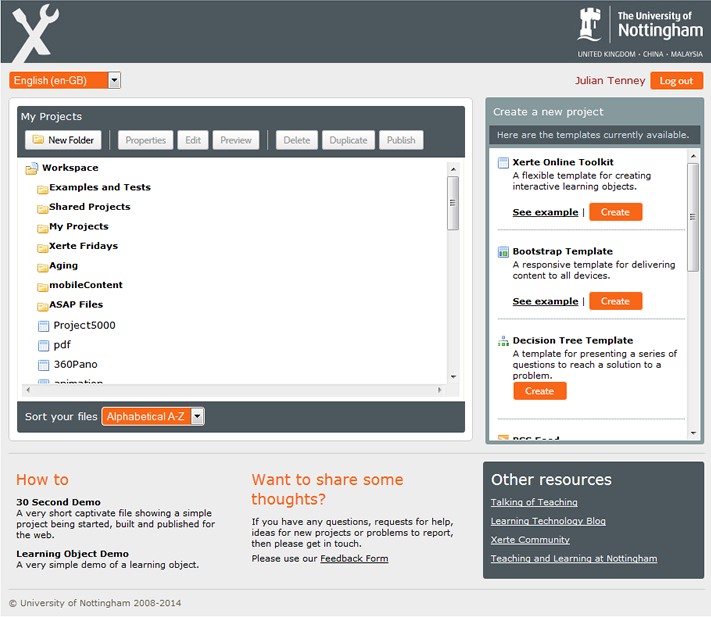The screenshot, taken from a student at the University of Nottingham, features a user interface with a light grey background. At the top, a charcoal grey rectangle spans the entire width of the image. On the far left of this bar, there are two emblems: a wrench and a wood chipper. On the far right, a castle tower icon is followed by the "University of Nottingham" written in white text. Directly beneath, the text "United Kingdom, China, Malaysia" is displayed.

An orange rectangle sits below this bar on the left, containing a drop-down menu labeled "English" in white text. Adjacent to it in red text is the name "Julian Tenney." To the right, another orange rectangle with white text reads "Log Out."

In the central portion of the screenshot, a large black rectangle featuring the text "My Projects" in white occupies the left side. Below this are multiple grey buttons labeled: "New Folder," "Properties," "Edit," "Preview," "Delete," "Duplicate," and "Publish." Further down the left column, various project and folder names such as "Workspace," "Examples and Tests," "Shared Projects," "My Projects," "Zerte Fridays," "Aging," "Mobile Content," "ASAP Files," "Project 5000," "PDF," and "360p ANO" are listed.

At the bottom of this column, the text "Sort Your Files, Alphabetical A-Z" and "How To's," "30 Second Demo," and "Learning Object Demo" are visible. To the right, a text box prompts, "Want to Share Some Thoughts."

On the right side, a prominent rectangle contains the option "Create a New Project." Below this rectangle, a list of currently available templates is displayed, including "Zerte Online Toolkit," "Bootstrap Template," and "Decision Tree Template." The bottom right corner features the text "Other Resources."